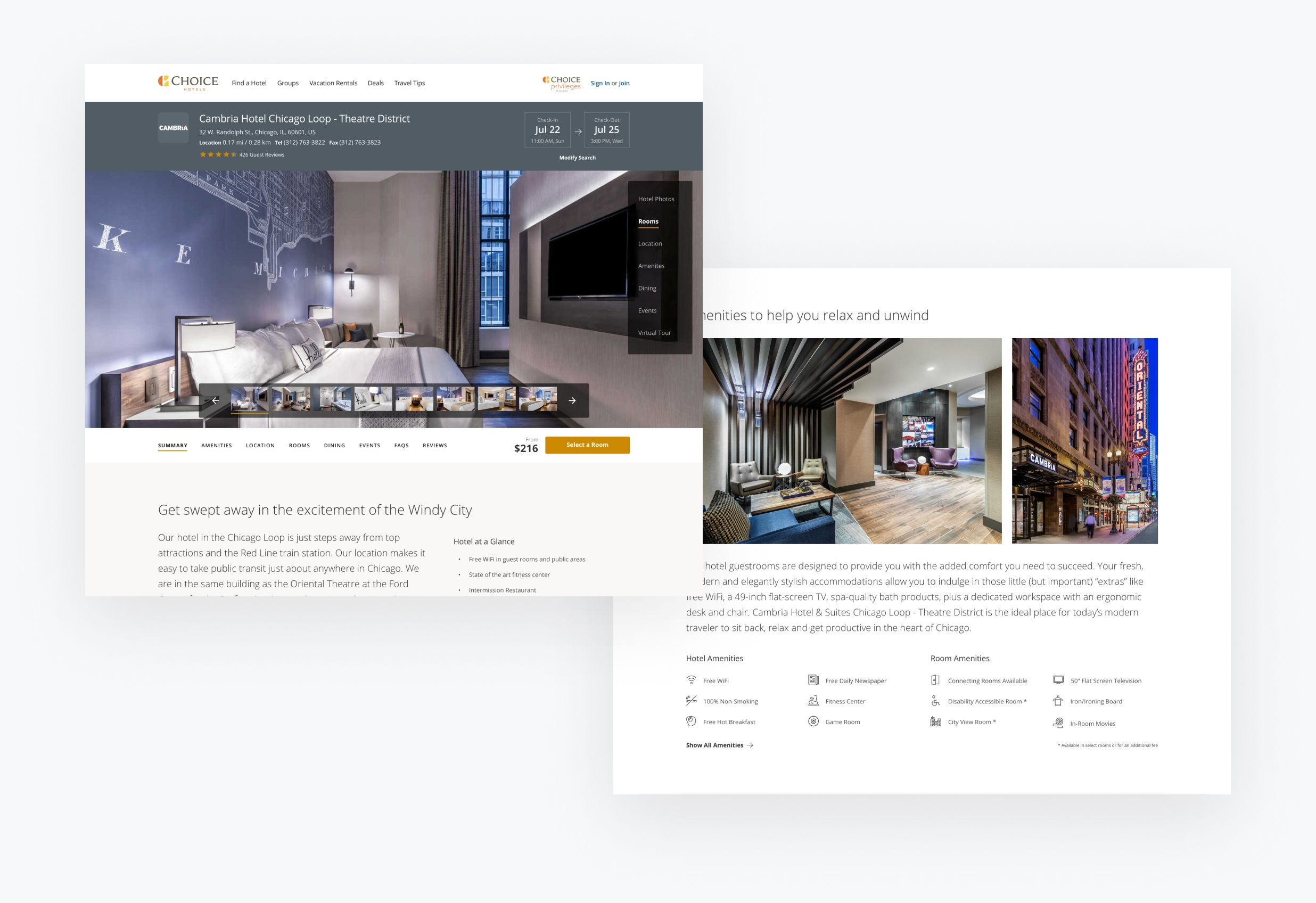The image depicts two distinct web pages overlaid on each other: one occupies the upper left section and the other the lower right corner. The upper left page is prominently labeled "Choice" accompanied by a gold symbol. It details a hotel located in the Chicago Loop, specifically in the Theater District, with a date range from July 22nd to July 25th. Below this information is a large photograph showcasing a spacious hotel room. The room features a large bed adorned with white pillows and covers, set against a blue wall decorated with a map and some text. A large flat screen TV is mounted on the wall in front of the bed. Underneath the photo, there is a paragraph of descriptive text accompanied by a gold button for further actions.

In the lower right section, the second web page displays two additional images: one depicts the interior of the room, while the other shows the exterior of the building. This section includes a brief paragraph of information and a series of four lines of different options available for selection.